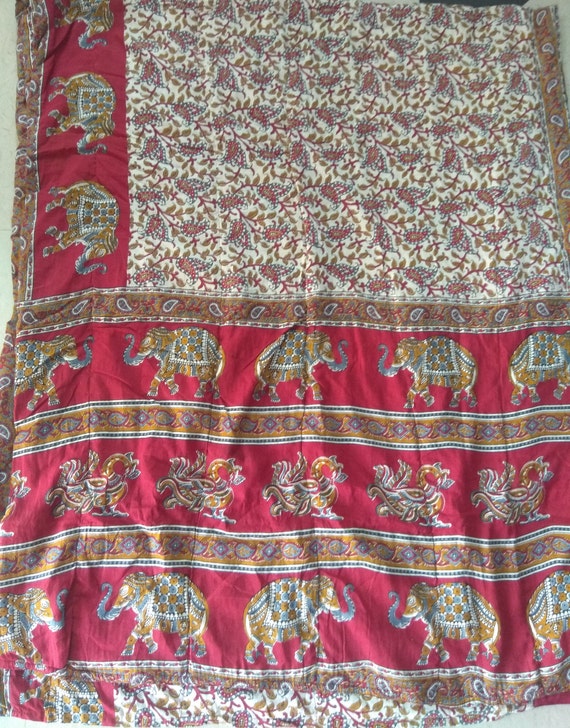In this detailed image of a quilt or blanket, we see intricate and colorful textile designs. Dominated by a rich red color, the fabric features three distinct sections. At the top, there are floral decorations with green leaves and red flowers. The middle section showcases golden-yellow elephants with grey trunks and blue accents, adorned with paisley patterns. These elephants appear to be in motion, taking confident steps forward. Below them, there are dynamic dragon shapes in brown, winged and appearing lively. The bottom section includes larger elephants, again predominantly golden-yellow, with ornate detailing. The quilt or blanket rests on a grey platform in the bottom right corner, accentuating its vibrant colors. This quilt's primary palette includes shades of red, brown, yellow, grey, and blue, intricately woven into a harmonious and visually striking textile piece.